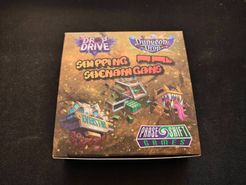The photograph depicts a small, square object, likely a box, with a gold-colored top, set against a dark, seemingly black background. The overall tone of the image features brown and beige hues with a slightly fuzzy quality. The box cover showcases intricate and unusual cartoonish graphics that appear to illustrate objects flying through space. The depicted objects are possibly spaceships or other fantastical entities with shades of green, pink, brown, blue, and purple.

Prominently displayed at the top of the box is the phrase "Drop Drive" written in a purple rectangle, and below it, foreign text which might be in an Asian language, featuring the word "Sanping". There is also a hard-to-decipher long word beginning with 'S'. This section of the box includes another label, which consists of an inverted purple triangle containing the words "Dungeon" and additional barely readable text.

In the lower right corner, there is a purple and yellow box with an open mouth and teeth, resembling a creature. There is also a three-dimensional rectangular bar with purple and green text mentioning "Shift Games".  The visual style and ambiguous familiar yet exotic language suggests it could be a packaging for a comic book, video game, or board game, marked by Asian-inspired and computer-type graphics, both fantastical and surreal. The dark, somewhat blurry photograph gives an intriguing, mysterious feel to the object depicted.